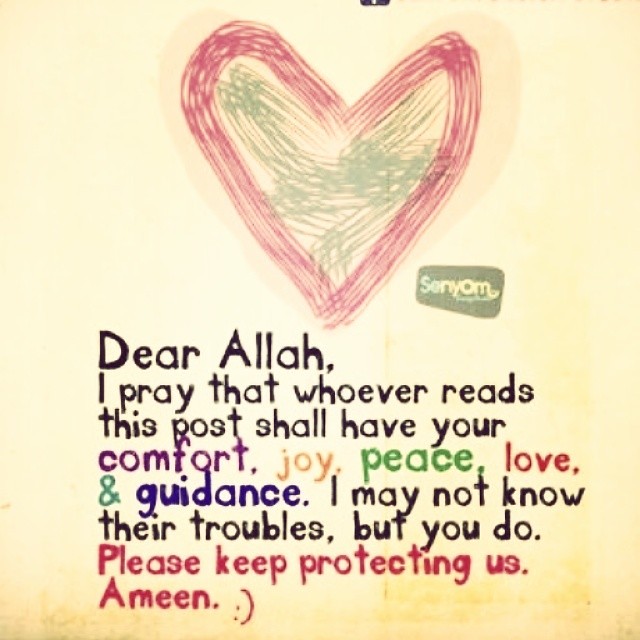The image depicts a hand-drawn artwork resembling a meme with a heartfelt prayer. Central to the image is a large heart, outlined in red and filled in with green, giving it a childlike, crayon-scribbled appearance. The heart sits on a faded yellow background, accompanied by text that reads:

"Dear Allah, I pray that whoever reads this post shall have your comfort, joy, peace, love, and guidance. I may not know their troubles, but you do. Please keep protecting us. Amen."

The words "comfort," "joy," "peace," "love," and "please keep protecting us" are color-coded in purple, yellow, green, red, and red respectively, adding emphasis and visual interest. Above the text, a small heart adds to the hand-drawn charm. Notably, the drawing features a small logo with white text inside a slanted black rectangle, spelling out "SONYOM." A smiley face sits next to the logo, further enhancing the whimsical, childlike feel of the image.